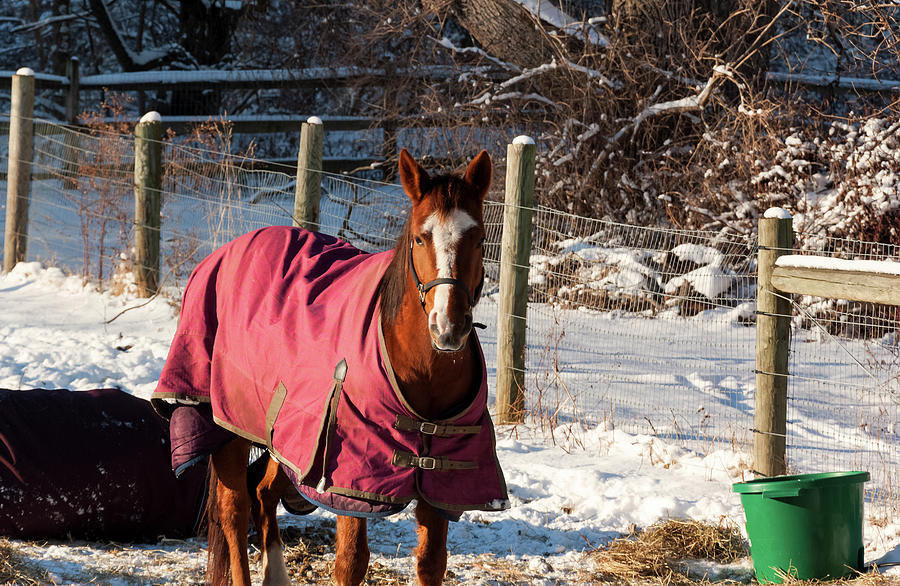In this detailed winter scene, a chestnut horse stands in a snowy, fenced-in field, its attentive gaze fixed on the camera. The horse is wearing a red coat with two brown straps and silver buckles in the front, providing extra warmth in the cold weather. A white stripe runs down the center of its face from its muzzle to its eyes. Beside the fence in the bottom right-hand corner, a green bucket sits on the ground, surrounded by patches of hay that contrast against the snow-covered terrain. The field is enclosed by rounded gray fence posts strung with chicken wire, forming a diagonal line toward the background. Beyond the fence, a serene winter landscape of snow-blanketed rocks, trees, and brush extends into the distance, highlighting the tranquil yet cold ambiance of the scene.